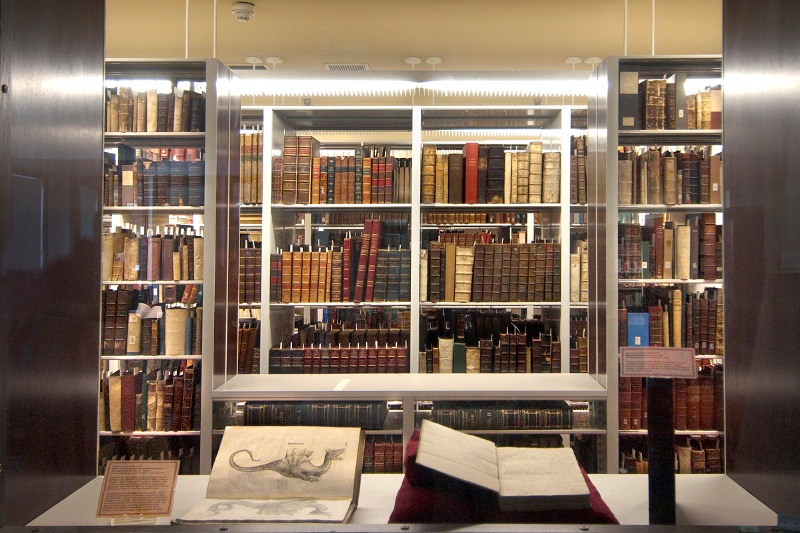The image captures an ancient and valuable library filled with shelves of old books of varying sizes and faded bindings, many marked with bookmarks or cataloging information. Prominently featured in front of these background shelves are two tall bookcases flanking a shorter central shelf, which houses large books that could be atlases, all indicating their considerable age. In the foreground, two open books rest on a small white shelf: the book on the left displays an illustration of a dragon or sea monster, while the one on the right is open to text. Descriptor cards lie next to each open book, likely providing further details about their contents. The ceiling above has a tan hue, adding to the historic ambiance of the scene.